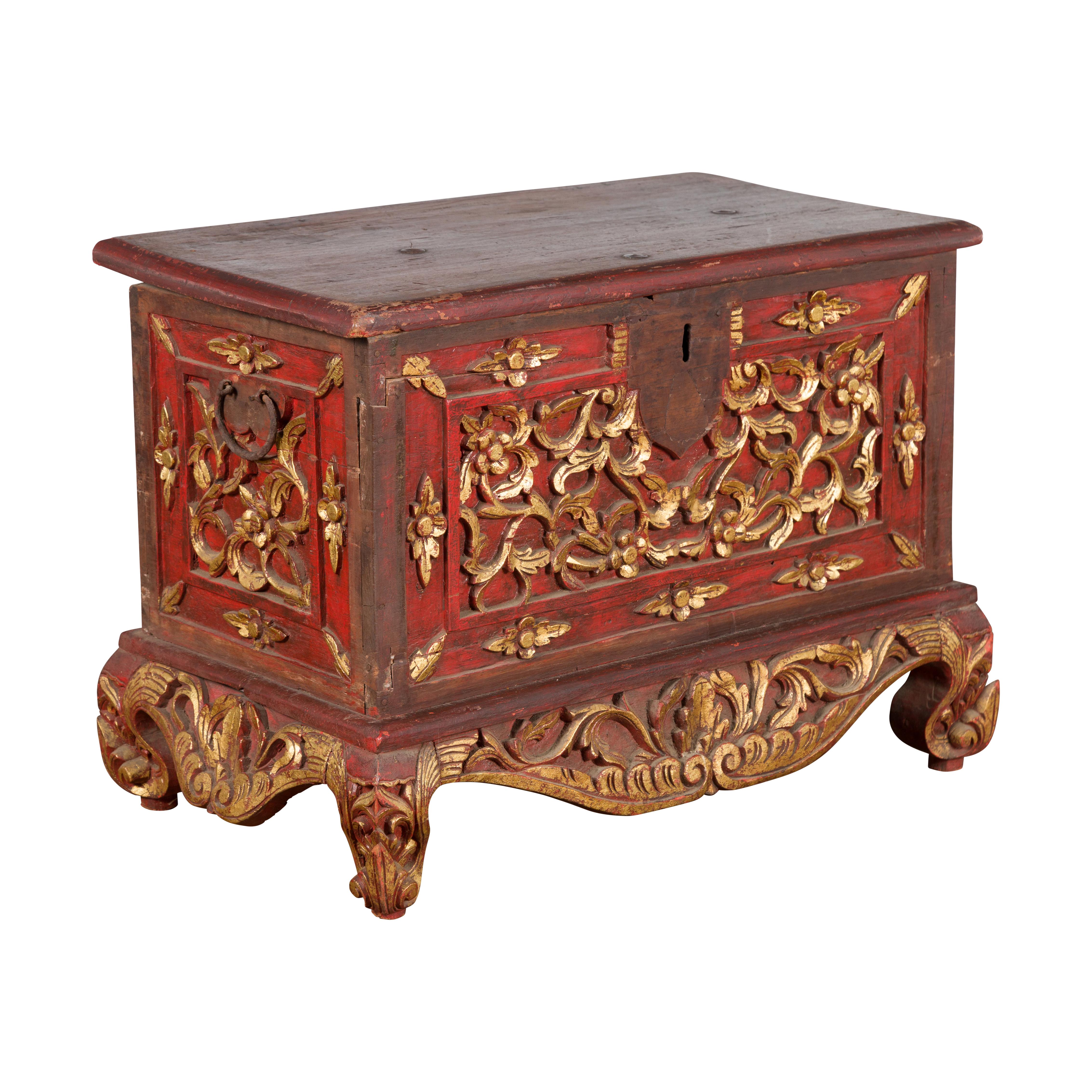This photograph captures an ornate, antique-looking chest that exudes a sense of historical elegance. The chest features a wooden top stained a rich, reddish-brown, contrasting with its red front. Both sides of the chest display a distinctive keyhole positioned within a shield-shaped brown area at the top front. The piece is rectangular in shape and includes handles on either side, crafted from thin metal, adding functionality to its decorative appeal. 

Gold or brass-colored decorative elements adorn both the front and the sides of the chest, highlighting its intricate craftsmanship. The bottom edge includes an elaborate apron-like area, featuring gold and brown carvings that appear to be inspired by plant motifs. The chest stands on short, intricately designed legs, which are curvy and reminiscent of clawfoot designs.

The overall appearance of the chest suggests it could be a treasured piece from the 1800s, possibly intended to store books, clothes, or shoes. With its worn and scuffed cherry-brown wooden surface, it carries the charm of an item that has been well-loved over the years. Set against a plain white background, the true scale of the chest is ambiguous; it might be a small jewelry chest or a larger trunk meant to sit at the foot of a bed.